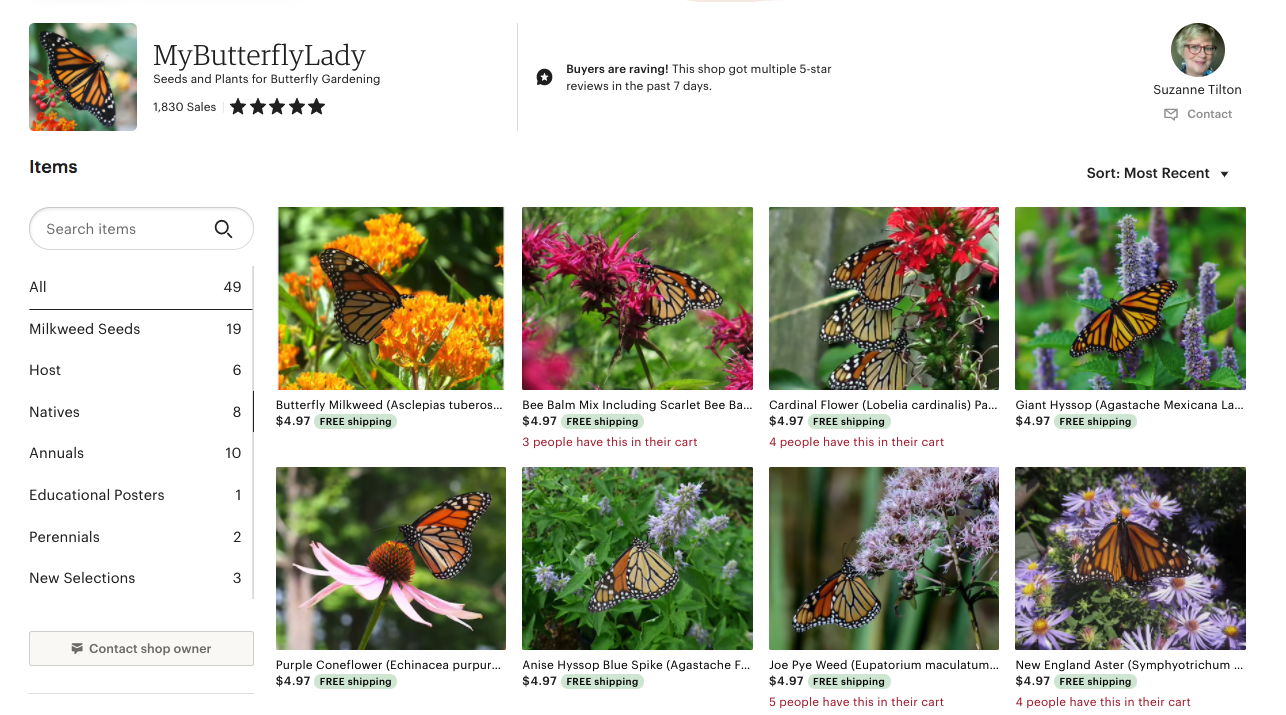A screenshot of a website titled "My Butterfly Lady: Seeds and Plants for Butterfly Gardening" is prominently displayed. The top left corner features a brand logo including a butterfly perched on flowers, accompanied by the store's details: "1,830 sales" and a 5-star rating. Directly below, a search bar and a menu for item categories include options such as "All (49)," "Milkweed Seeds (19)," "Host (6)," "Natives (8)," "Annuals (10)," "Educational Posters (1)," "Perennials (2)," and "New Selections (3)." A "Contact Shop Owner" button sits at the bottom of the menu.

To the right, a banner touts the shop's stellar reputation with the phrase, "Buyers are raving! This shop got multiple 5-star reviews in the past 7 days." The top right corner features the shop owner, Suzanne Tilton, with her photo directly below her name, alongside a message icon labeled "Contact." Below this, a sort menu is open to "Most Recent."

The primary section of the page showcases eight distinct product listings for butterfly-attracting plants, each priced at $4.97 with free shipping. The offerings include:
1. Butterfly Milkweed
2. Bee Balm Mix (description partially cut off)
3. Cardinal Flower (Lobelia cardinalis) with 4 people having it in their cart
4. Giant Hyssop, with its technical name provided
5. Purple Coneflower
6. Anise Hyssop (Blue Spike variety)
7. Joe Pye Weed
8. New England Aster

Each product image displays the specified flower with a Monarch butterfly on it, enhancing the inviting visual appeal for prospective buyers.